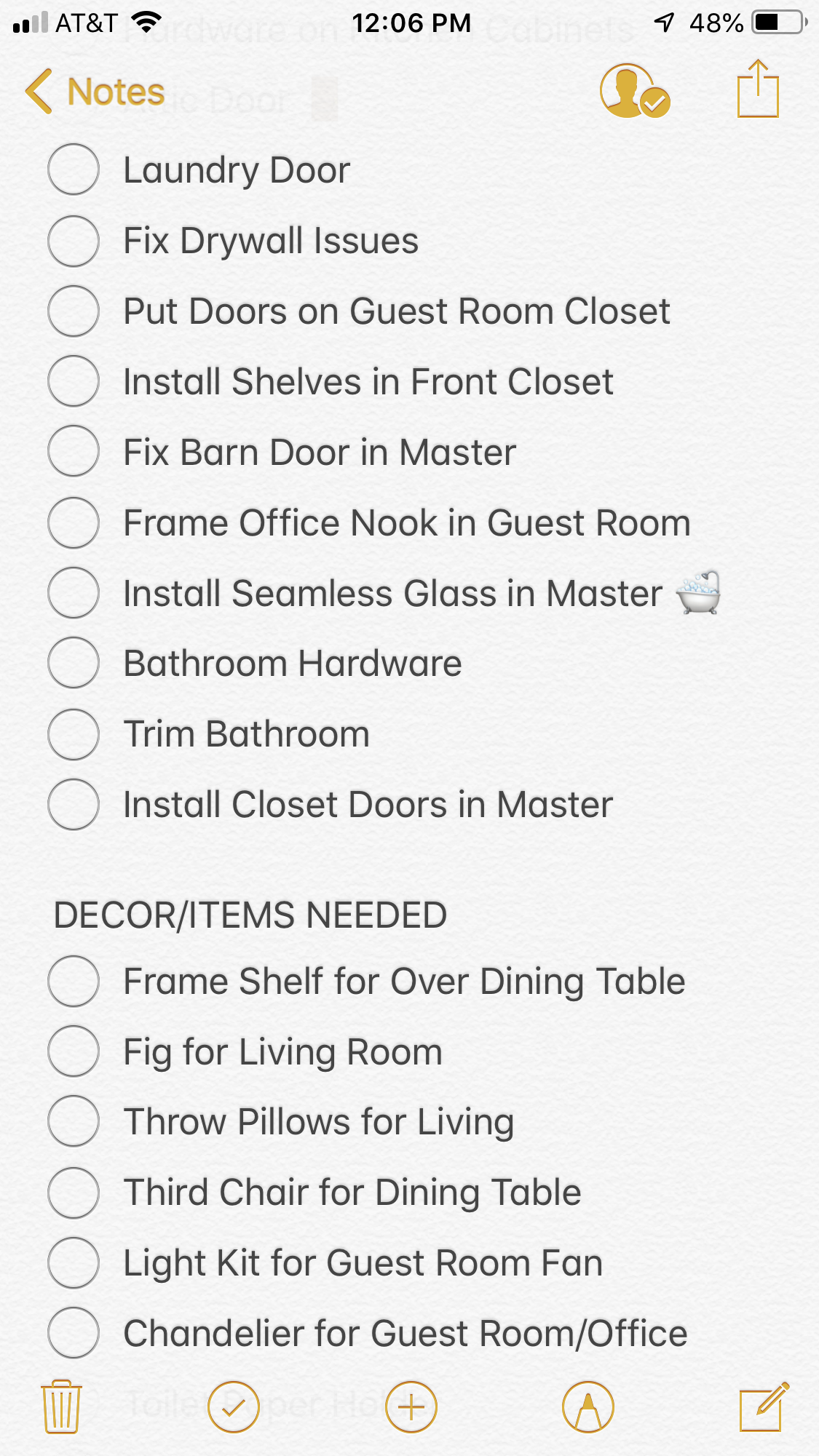This is a detailed screenshot from the Notes app on a mobile phone. At the top of the screen, the notifications bar displays the time as 12:06 p.m. centrally, with a 48% battery icon on the top right, and an AT&T signal icon on the left. Below the notifications bar, the app's name "Notes" appears in gold on the left, accompanied by a gold silhouette avatar with a check mark and what appears to be a share button on the right.

The content of the note is organized into two sections, each with a list of tasks or items. The first section lists ten tasks related to home improvement:

1. Laundry Door
2. Fix Drywall Issues
3. Put Doors on Guest Room Closets
4. Install Shelves in Front Closet
5. Fix Barn Door in Master
6. Frame Office Nook in Guest Room
7. Install Seamless Glass in Master
8. Bathroom Hardware
9. Trim Bathroom
10. Install Closet Doors in Master

The second section, titled "Decor / Items Needed," includes six items:

1. Frame Shelf for Over Dining Table
2. Fig for Living Room
3. Throw Pillows for Living
4. Third Chair for Dining Table
5. Light Kit for Guest Room Fan
6. Chandelier for Guest Room / Office

At the bottom of the screen, the footer features five icons for various app functions: a trash icon on the left, a check icon, a plus icon in the middle, a marker icon, and a notepad icon on the bottom right corner.